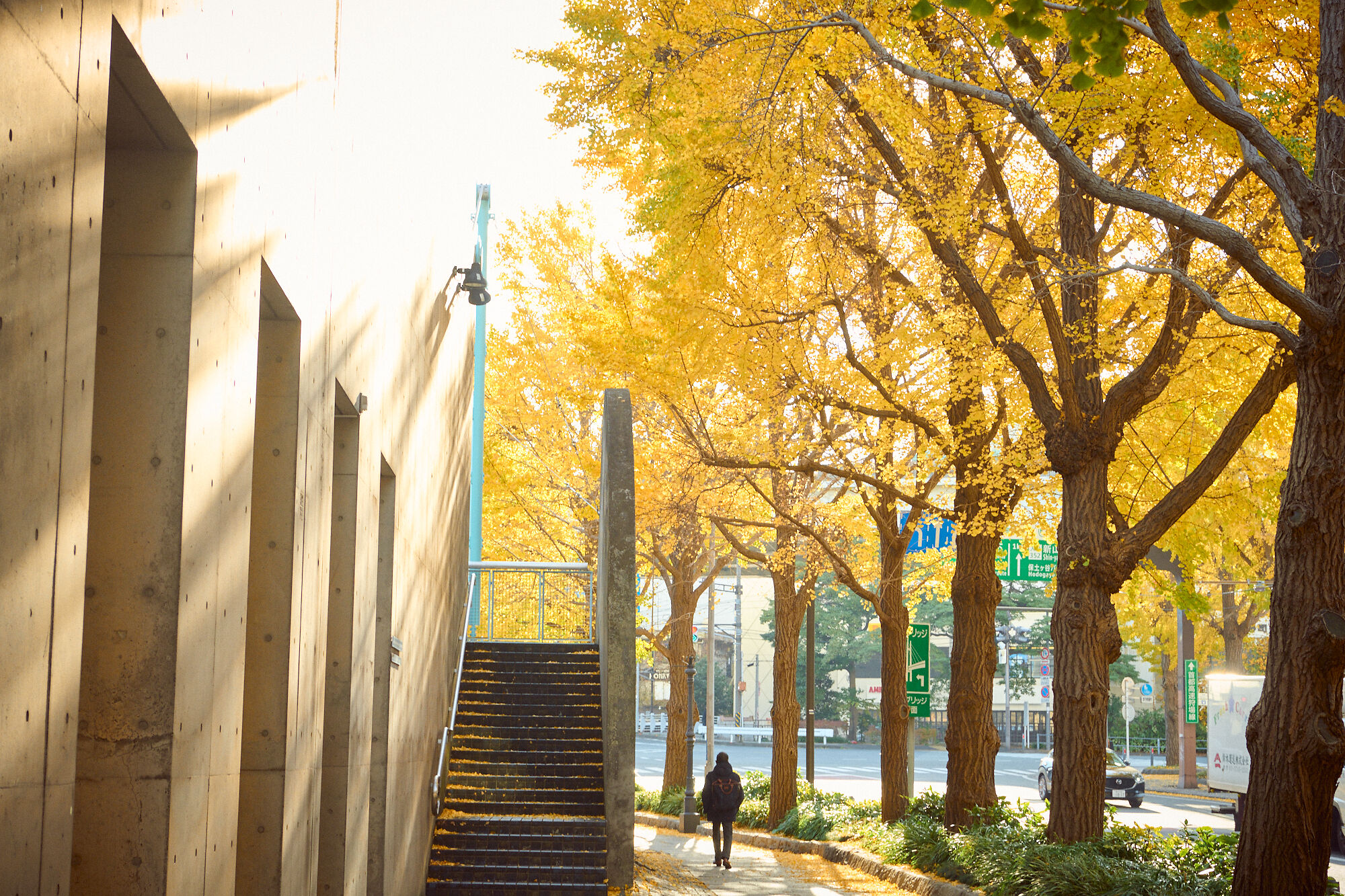In this vibrant fall city scene, a concrete building dominates the left side of the photograph. The building features several tall, rectangular doorways and is approached by a set of concrete steps. The sidewalk next to the building leads towards a landscaped area adorned with mature trees showcasing bright yellow leaves. A man dressed in winter wear, consisting of a long black coat and black pants, is seen walking down the sidewalk. The sun shines through the trees, casting light onto the building, enhancing the warm autumn ambiance. On the right, in the far background, street signs and cars driving on a road are visible, adding to the urban atmosphere. Above, two floodlights are mounted to illuminate the stairs, though they remain off in the daylight.